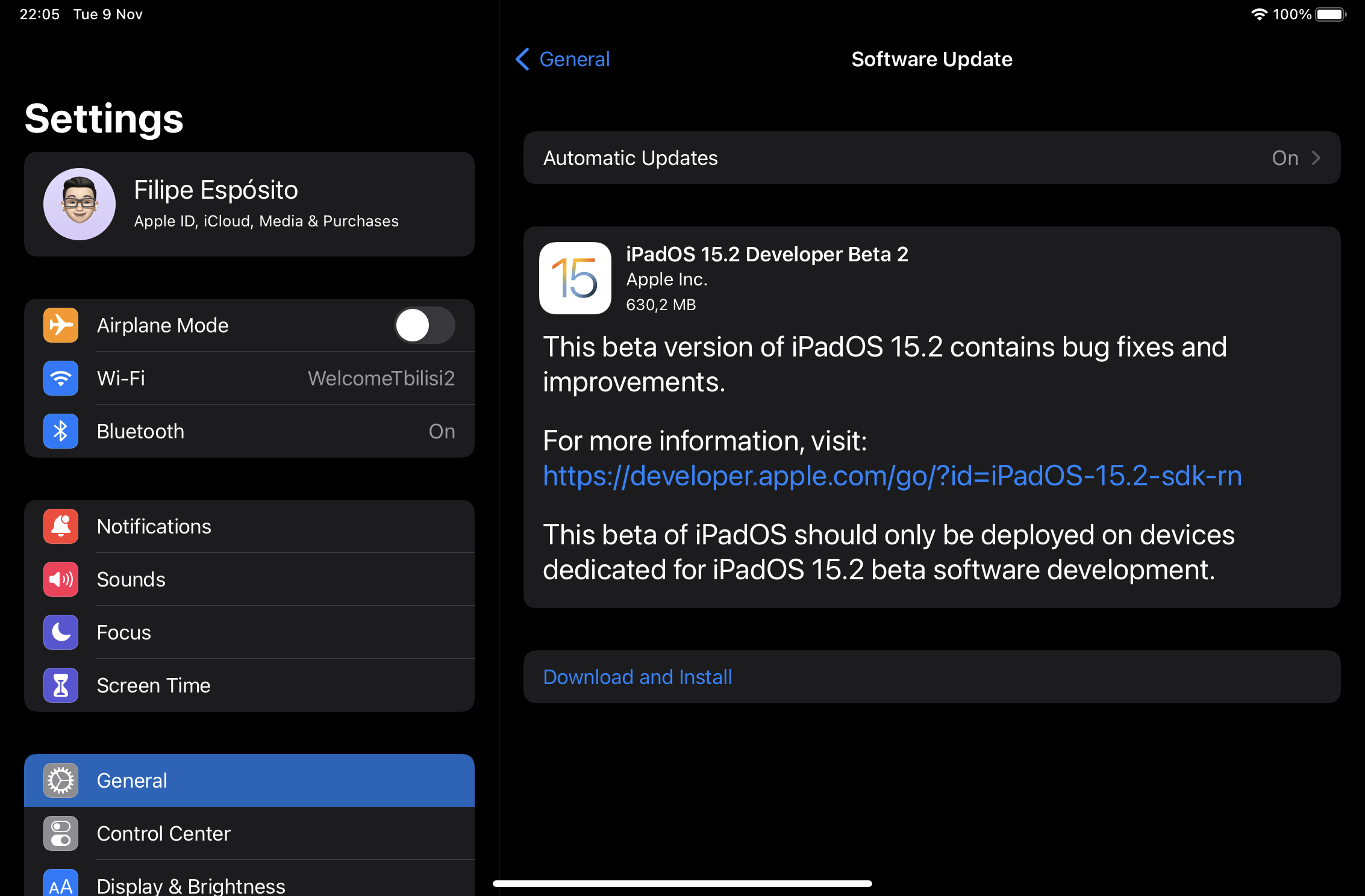The image depicts a smartphone settings screen with a sleek black background. At the top left corner, the screen displays the time as 22:05 on Tuesday, November 9th. On the top right corner, the Wi-Fi signal icon is visible alongside an indicator showing 100% battery remaining.

On the left side, a prominent heading in white reads "Settings". Directly below this heading is a small icon beside the name "Philippe Esposito". Underneath Philippe's name, a series of grouped icons and titles are displayed, representing various functionalities.

In the first grouping, the functionalities include:
1. An orange airplane icon labeled "Airplane Mode".
2. A blue Wi-Fi icon labeled "Wi-Fi".
3. A Bluetooth icon labeled "Bluetooth" indicating that it is currently enabled.

In the second grouping, the following functionalities are listed:
1. A bell icon labeled "Notifications".
2. A speaker icon labeled "Sounds".
3. A moon icon labeled "Focus".
4. An hourglass icon labeled "Screen Time".

Below these groupings, the "General" option is selected. On the right side of this section, details about a software update are shown. It advises that automatic updates are currently configured to be on. Additionally, it mentions the availability of a beta version of iPod OS 15.2 with some improvements, along with a "Download and Install" button positioned beneath these details.